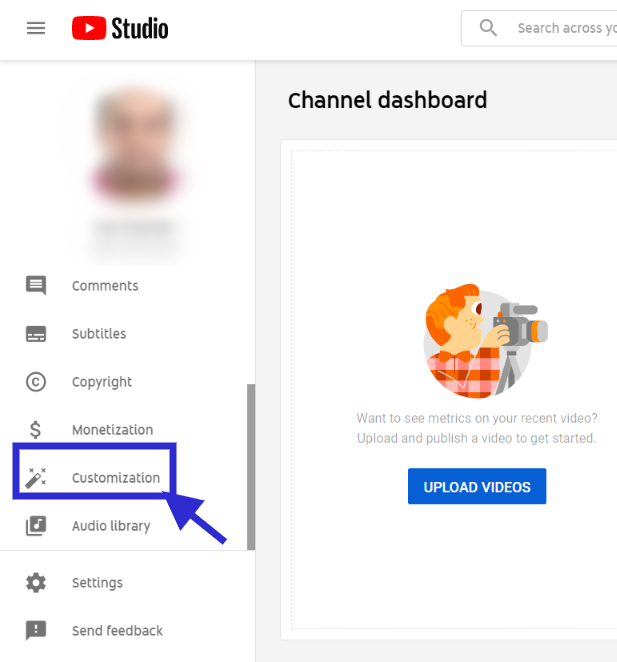The image depicts a partial view of the YouTube Studio dashboard menu. The prominent YouTube logo is followed by the term "Studio" at the top. Below, a list of several options starts with "Channel Dashboard" and includes "Comments," "Subtitles," "Copyright," "Monetization," and "Customization." The "Customization" option is notably highlighted with a blue square, and an arrow points toward it, suggesting an interest in customization settings.

To the right, a blue-highlighted button with white text reads "Upload Videos." Accompanying this is an illustrated image of a person with red hair wearing a plaid shirt, holding a camera aimed outward. Beneath this illustration, there is a prompt that reads, "Want to see metrics on your recent video? Upload and publish a video to get started."

On the left side, where the main menu options are, there is also a blurred-out photograph of a person at the top, likely representing the user's profile. The entire interface is set against a clean white background, emphasizing the different dashboard elements.